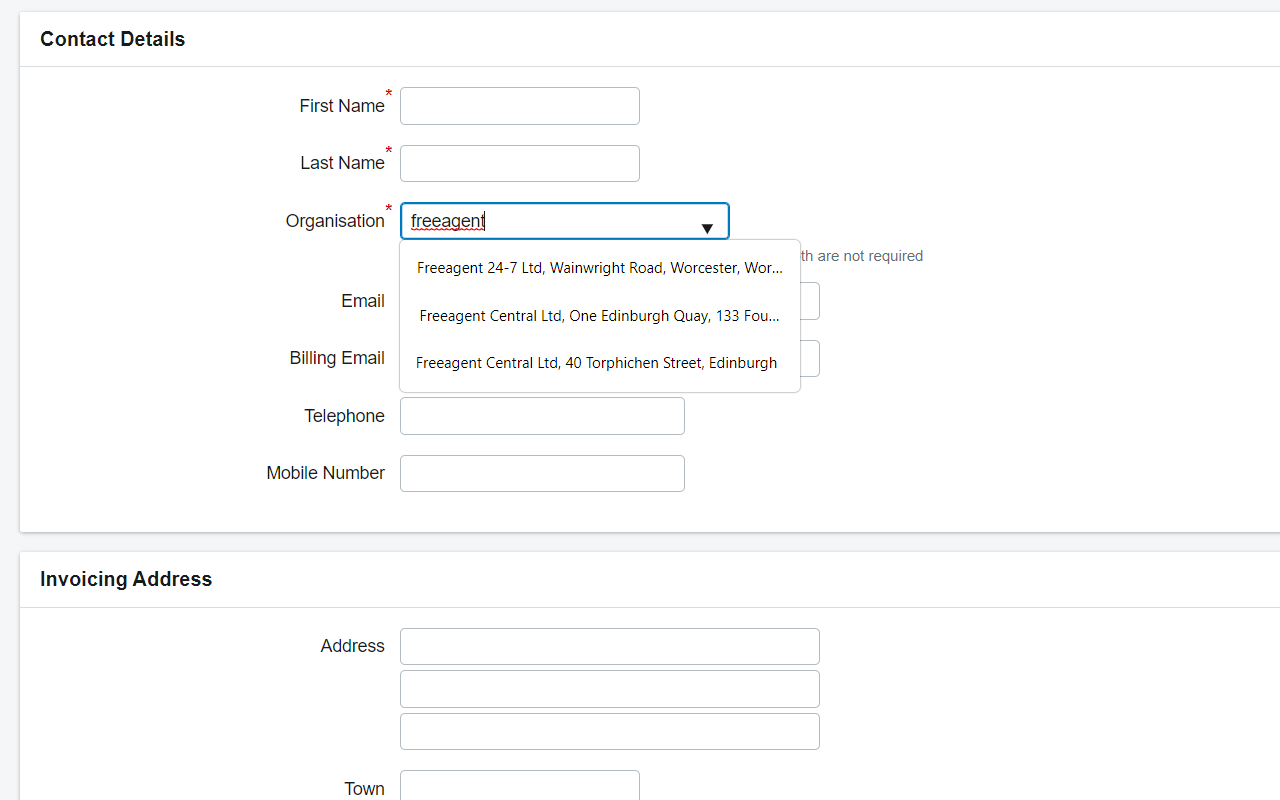The image is a screenshot of an online form with a predominantly white background. The layout features a very pale gray border at the top and along the left side, but no border on the bottom. A light gray line separates the upper and lower sections of the form.

The top half of the form is focused on "Contact Details," which is left-aligned in black text in the upper-left corner. A thin, pale gray line runs horizontally beneath this title. Below this, the form is indented, creating a significant amount of white space on the left side before the input fields begin. 

The input fields include:
1. **First Name**: A text box for entering the first name, indicated by a red asterisk, signifying it is a required field.
2. **Last Name**: A text box for entering the last name, also marked with a red asterisk as a required field.
3. **Organization**: Displayed with British spelling ("Organisation"), this field features a drop-down menu. The user has begun typing "Free Agent," causing the drop-down menu to display three selectable options. This menu overlaps the subsequent text boxes.

Following the drop-down menu are fields for:
- **Email**
- **Billing Email**
- **Telephone**
- **Mobile Number**

Notably, these fields do not have red asterisks, implying they are not mandatory.

A pale gray band serves as a divider before the form transitions to the "Invoicing Address" section. This section mirrors the indent seen above and includes fields for:
- **Address**: Three blank lines are provided for the full address.
- **Town/City**
- **Postcode**

The lower part of the form is cropped off, but there are likely additional fields for completing the address details.